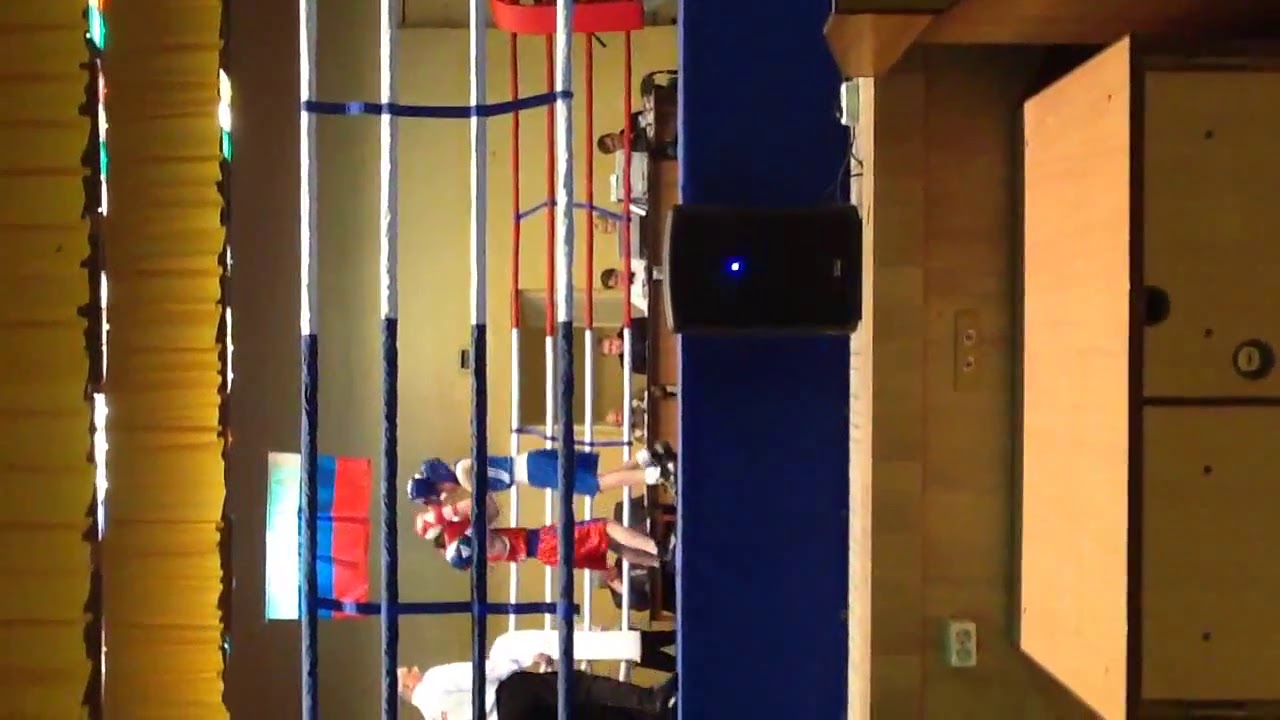In this sideways photograph of an indoor boxing match, two young fighters are engaged in the ring. The fighter on the left is wearing blue trunks, a blue shirt, and a matching blue helmet, while the fighter on the right is dressed in red trunks and red gloves, although their helmet is not visible. Both are under the watchful eye of a referee clad in a white shirt and dark pants. The boxing ring features ropes that are half white and half dark blue. In the background, a beige wall is adorned with the Russian flag, displaying horizontal stripes of white, blue, and red. Above the scene, a yellow ceiling is visible. The overall ambiance of the arena is further characterized by a mix of blue, white, and red colors, along with a distinctively noticeable beige wooden cabinet and a silver outlet on the right-hand side.